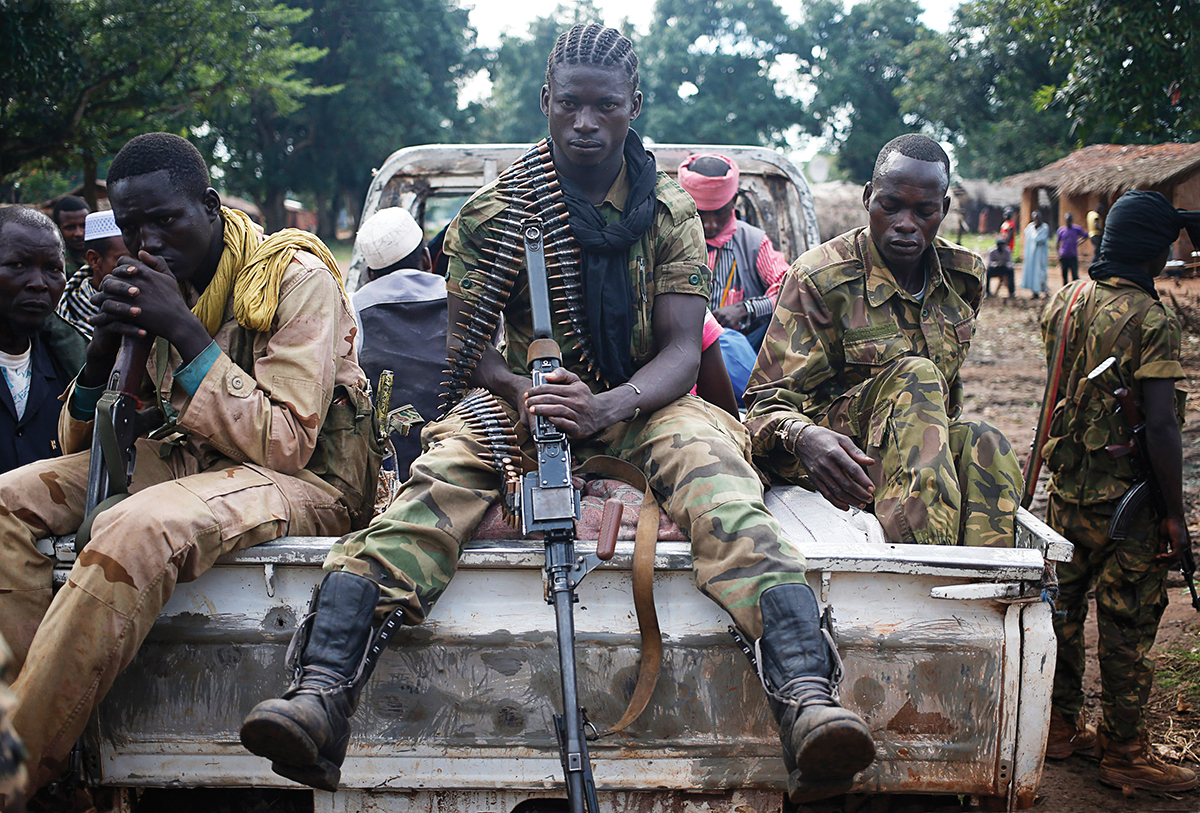The image vividly captures a scene of apparent African soldiers, three of whom are prominently seated in the back of a weathered, white pickup truck on a dusty village road. These soldiers, all black males, appear to be aged between their late teens and thirties. Each is donned in various styles of camouflage army gear, with the man on the left notably clad in a faded brown and pink uniform, while the other two wear matching tan camouflage uniforms. The central figure, who features cornrows, distinctively holds a machine gun and a bandolier of bullets draped across his chest, his feet dangling off the truck. The soldier on his left, with a headscarf concealing part of his face, grips an AK-47, similarly sitting with his feet hanging from the vehicle. The man on the far right, weaponless, sits with his feet tucked inside the truck. Additionally, two more individuals, possibly civilians or other soldiers, are seen in the truck bed – one with a red bandana and blue pants, the other in a black shirt with a traditional Muslim cap turned away from the camera. The scene is further animated by a variety of villagers adorned in colorful attire standing beside the road and by a hut and trees that complete the rural backdrop.